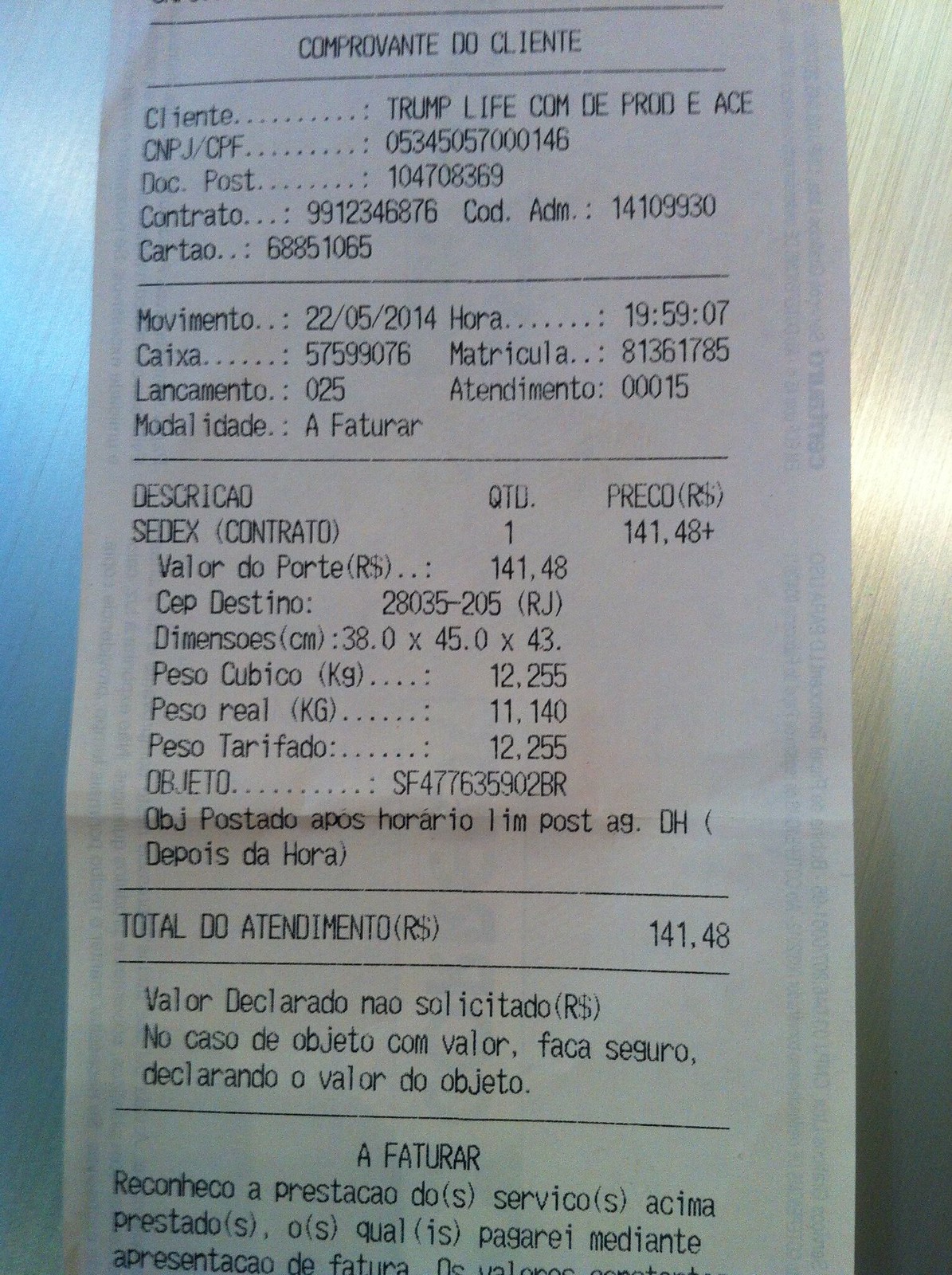This image features a white receipt prominently displayed on a flat, textured surface. The background is awash with a gradient of blue light on the left and white light on the right, creating a striking contrast. The gray surface beneath the receipt is adorned with skewed, vertical polishing lines that are darker than the base color, adding depth and interest to the scene.

The receipt itself stands out due to its crisp whiteness. At the top, text in Spanish reads "Comprobante del Cliente," indicating it is a customer's receipt. Directly below this, the receipt contains detailed client information, contact details, and a list of purchased items. The meticulous arrangement and lighting enhance the visual appeal, transforming a simple receipt into a striking subject.